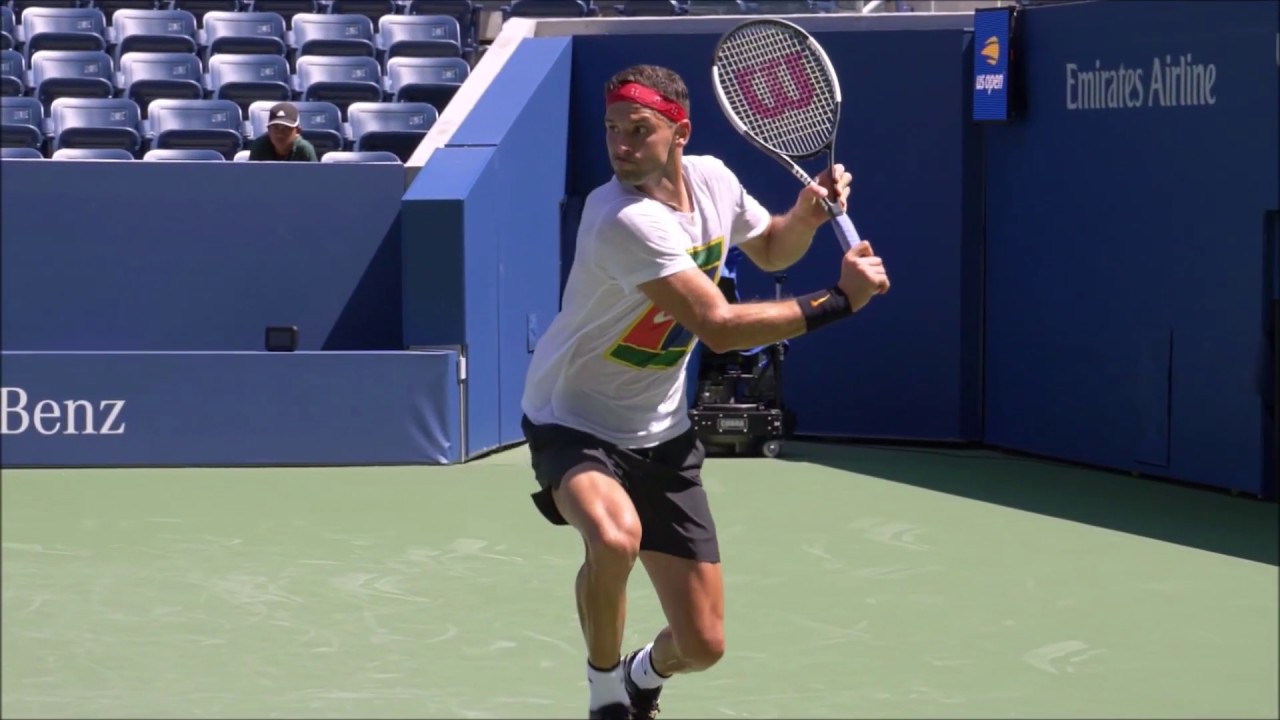The image captures a moment during a tennis match featuring a youngish male player, possibly in his 30s, with dark skin and brown hair. He's poised in a stance, ready to hit a ball with his blue and white tennis racket, which has a prominent "W" logo. The player is dressed in a white t-shirt with an unclear design, black athletic shorts, white socks, and black tennis shoes. He also sports a red headband and a black wristband on his right wrist. The green tennis court contrasts with the blue seats and navy blue wall in the background, which displays the "Emirates Airline" logo to the right. One spectator, wearing a green shirt and a mainly black hat with a white logo and outline, can be seen sitting in the blue seats on the left side, attentively watching the match. The player’s face shows intense concentration, highlighting his readiness to engage with the ball coming from the other side of the net.